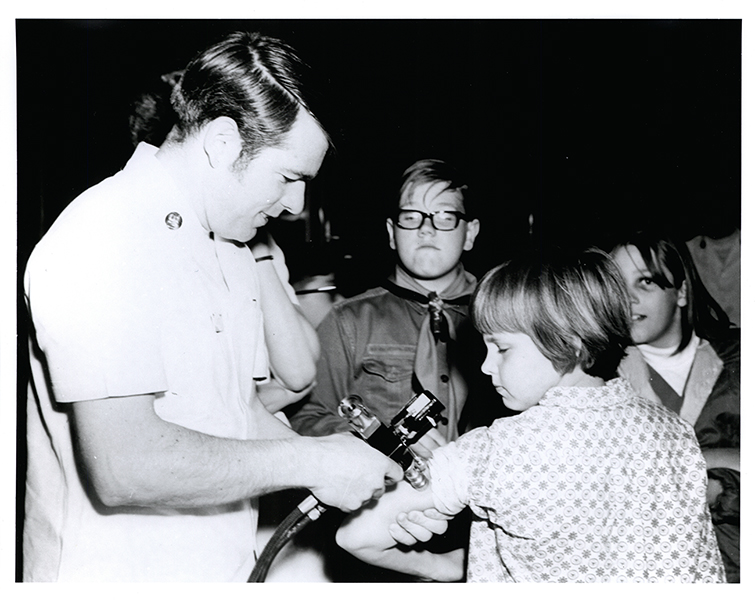In this vintage black-and-white photograph, a man, possibly a doctor or medical professional, is administering vaccines to children using a specialized vaccine gun. He is dressed in a short-sleeved white shirt and holds the device, which has two tubes extending from its bottom, against the left arm of a young girl who appears to be in elementary school, likely around first or second grade. The girl, with her light-colored, above-shoulder-length hair, looks down at the device with a slightly annoyed or upset expression, understandable given the medical context. Her shirt sleeve is rolled up to allow access to her arm. Standing nearby, a boy in a Boy Scout uniform watches the procedure attentively. He is light-skinned, wears dark-framed glasses, and has bangs falling over his forehead. The background is predominantly dark, adding contrast to the focused scene of the medical procedure.